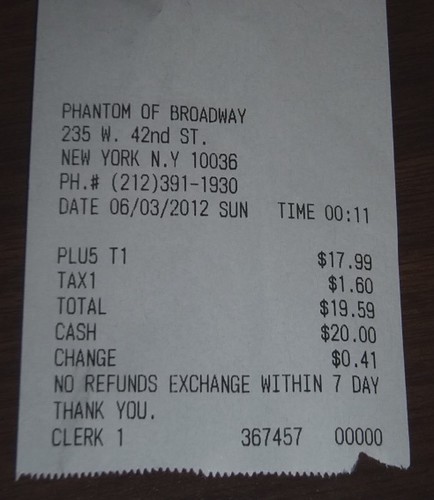The image depicts a detailed photograph of a light gray paper receipt, laying on a wooden surface. The text is black on a white, rectangular paper printout. At the top, the receipt reads "Phantom of Broadway," followed by the address "235 West 42nd Street, New York, NY 10036." Below, there is a phone number listed as "(212) 391-1930." The receipt is dated "06/03/2012," specifically a Sunday at "00:11." The purchase details show an item costing "$17.99" with an additional tax of "$1.60," bringing the total to "$19.59." The payment was made with "$20.00" in cash, resulting in a change of "$0.41." The receipt clearly states "No refunds. Exchange within 7 days. Thank you." The transaction was processed by clerk ID number "1-367-457-0000." The receipt is bordered by a dark gray outer background.